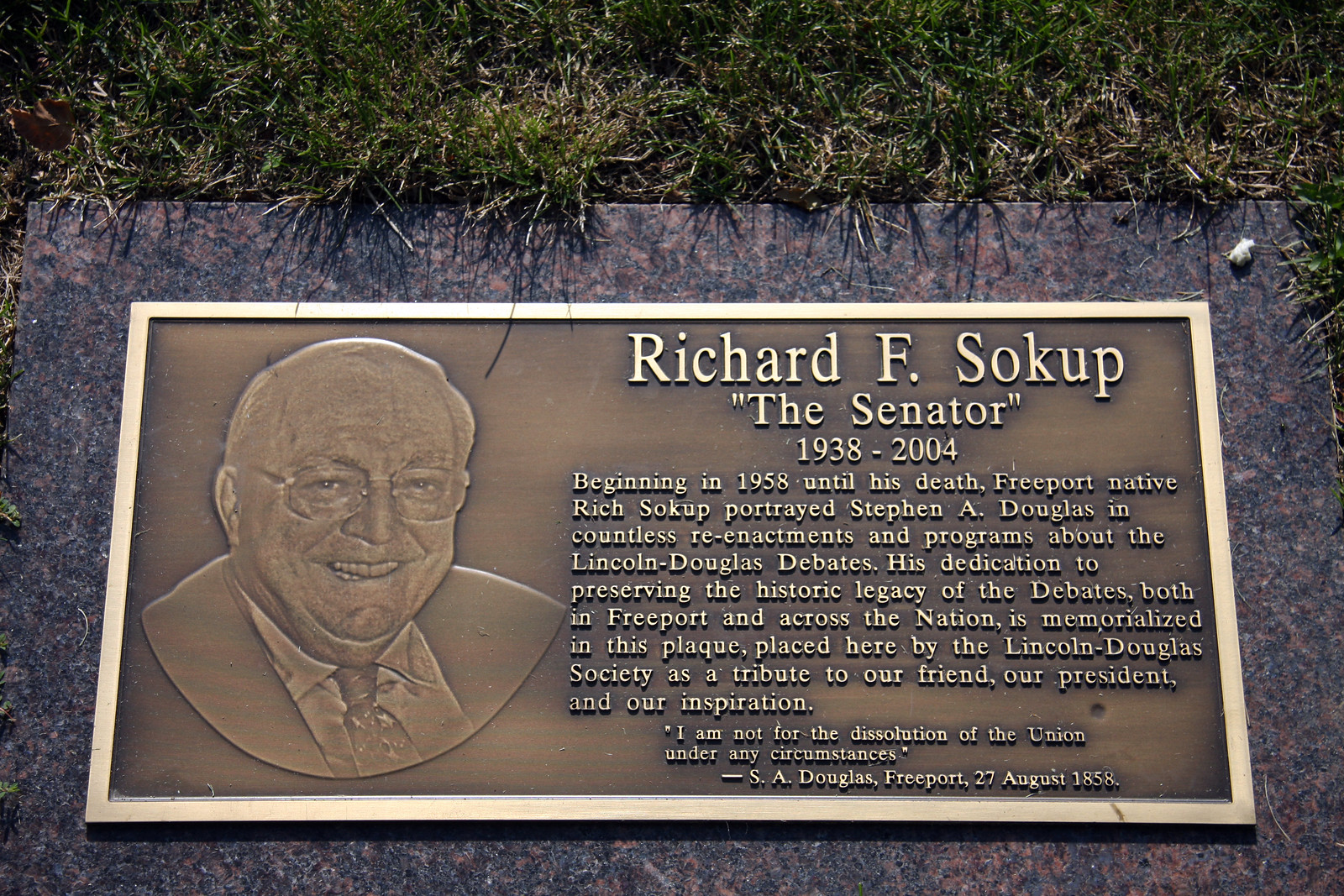The image depicts a memorial plaque embedded in a red granite stone, which lies flat on the ground amid a backdrop of grass. The plaque itself might be made of bronze or another metal and features an engraved portrait of an elderly man smiling, clad in a suit, tie, and glasses. The text reads "Richard F. Sokup 'The Senator' 1938-2004." A detailed inscription follows: "Beginning in 1958 until his death, Freeport native Richard Sokup portrayed Stephen A. Douglas in countless reenactments and programs about the Lincoln-Douglas debates. His dedication to preserving the historic legacy of the debates, both in Freeport and across the nation, is memorialized in this plaque, placed here by the Lincoln-Douglas Society as a tribute to our friend, our president, and our inspiration." While the plaque may appear to be part of a gravestone, it could also be a dedicated memorial placed by the Lincoln-Douglas Society, potentially situated in a park or another public space honoring his contributions.